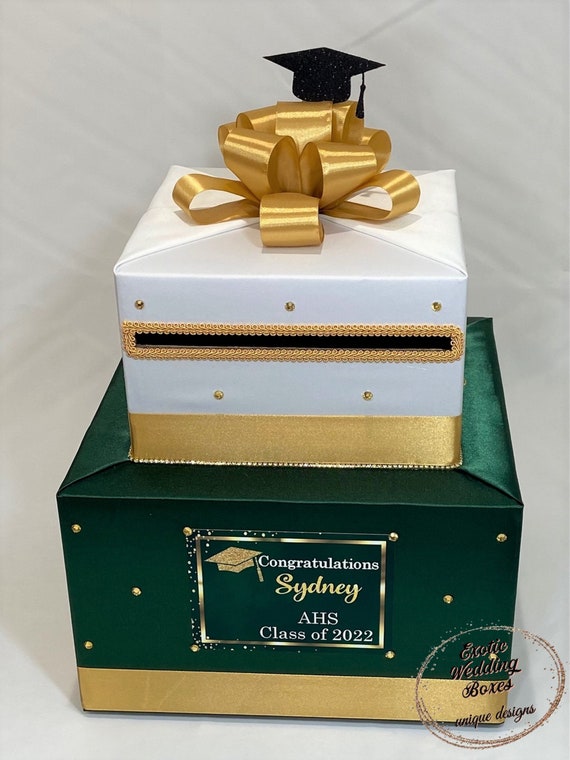This is a photograph of a uniquely designed graduation gift box intended for party attendants to drop their greeting and money cards. The structure consists of two stacked boxes with elegant gold accents. The bottom box is a satin dark green fabric with gold trim and is adorned with gold dots. It features a square that reads, "Congratulations Sydney AHS Class of 2022." The upper, slightly smaller white box also has gold trim and includes a slot for card insertion, framed by a gold fabric outline. Atop the white box, there is a gold bow, which is crowned by a small black, sparkly graduation cap. In the bottom right corner, there's a circular watermark that reads "Exotic Wedding Boxes, Unique Designs," indicating the origin or design inspiration of the item.